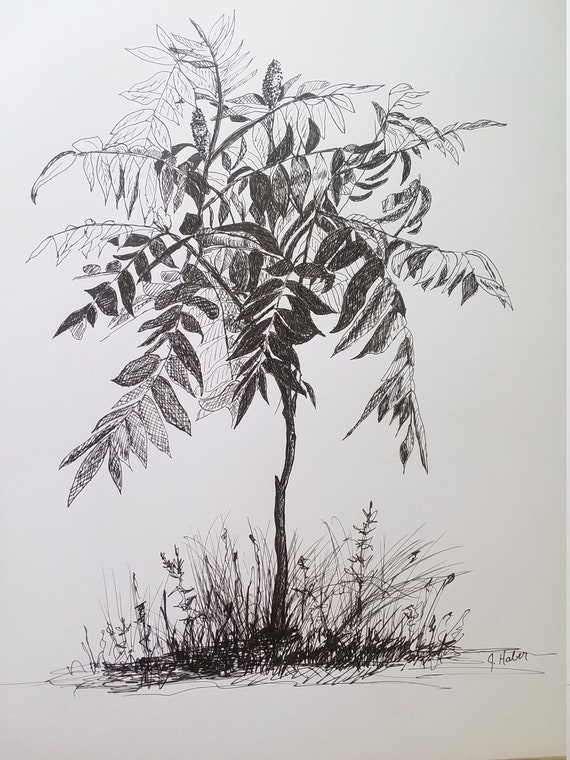This hand-drawn image, executed in dark pencil on an off-white or creamy white construction paper, depicts a small, bushy tree appearing about two inches in height. The tree is characterized by a delicate, thin trunk that gives rise to numerous branches covered in elongated, oval leaves. These branches, especially the lower ones, hang down due to the weight of the leaves. At the base of the tree, wild, unruly grass grows tall, enveloping the tree's roots and lower trunk. The leaves show varied shading, with those at the bottom being fully shaded and darker, indicating denser foliage, while the leaves at the top are lightly sketched, allowing the background to be visible through them. This intricate shading might suggest the direction of sunlight, enhancing the three-dimensional effect. In the right corner of the drawing, the artist’s signature, "J. Hallen," is visible.